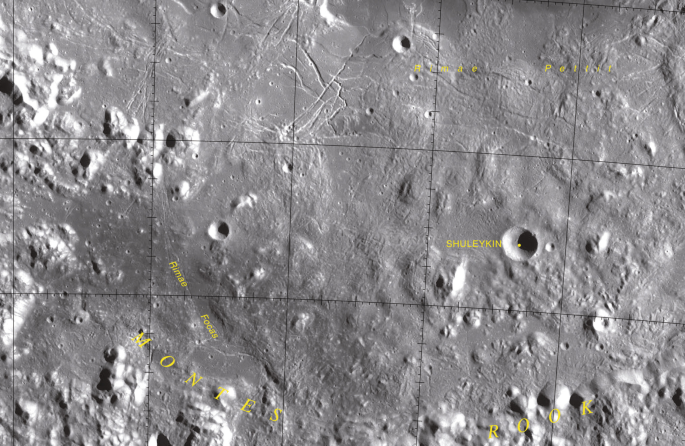The image depicts a detailed, black-and-white close-up of a gray surface resembling the moon, covered with numerous small craters and rugged, rock-like formations. The surface appears uneven, with raised rough patches on the left and more prominent rock-like structures on the bottom right. Scattered throughout the image are various yellow labels, including notable ones like "Montez Rook" and "Shoelaken." The perspective suggests the image was taken from above, likely reminiscent of satellite imagery. Black square outlines are also visible across the surface, adding to the detailed and mapped appearance of the moon-like terrain.